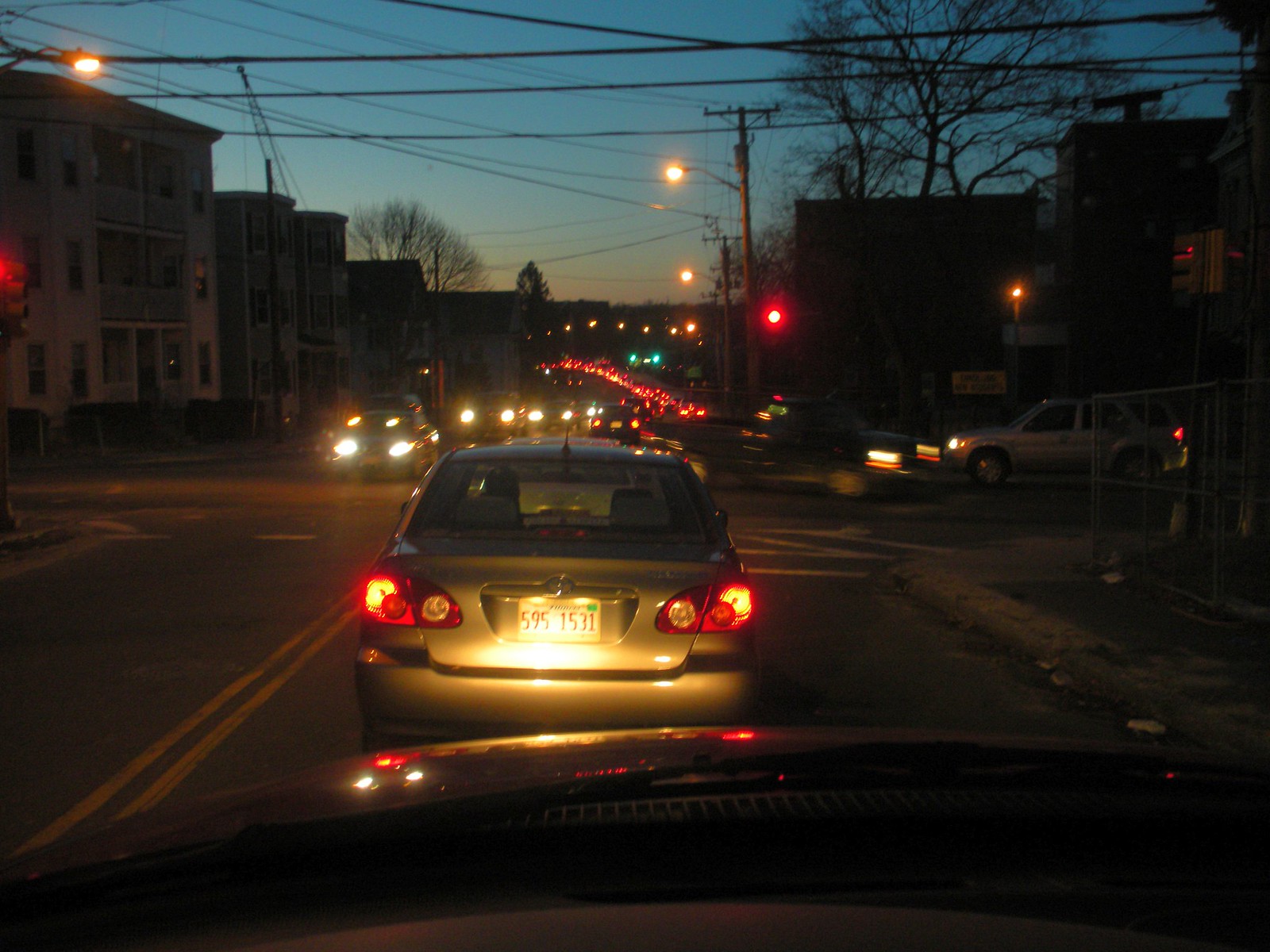A driver’s perspective shows a bustling four-way stop intersection. In front of the grayish-green sedan, a dark truck is making a left turn. Traffic can be seen on both sides, with a white SUV pausing at a stop sign across the intersection. Multiple cars are stopped on the opposite side, patiently waiting for their turn to proceed. The street is flanked by apartment buildings on both the left and right sides, bordered by a chain-link fence. An electronic crosswalk sign is also visible, emphasizing the urban setting of the scene.